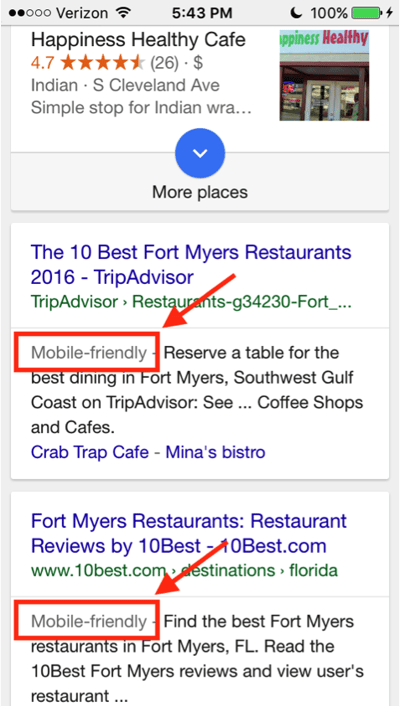This is a detailed screenshot from a smartphone displaying a list of restaurants in Fort Myers, Florida. The image is in a vertical rectangular format and shows various details from the phone's interface. In the top left corner, it indicates that the phone is using Verizon for its cellular signal and is connected to Wi-Fi. The time is displayed as 5:43 PM, and the battery icon shows a full 100% charge.

The image highlights several restaurant listings obtained from a search. One notable restaurant is "Happiness Healthy Cafe," which features a rating of 4.7 stars based on 26 reviews and has a single dollar sign, indicating a relatively affordable price range. This cafe is described as an Indian food establishment located on South Cleveland Avenue, though the description cuts off with the phrase "Simple Stop for Indian."

Other elements in the screenshot include references to "The 10 Best Fort Myers Restaurants 2016" from TripAdvisor, indicating a list or guide to top dining establishments in the area. Additionally, there is an entry titled "TripAdvisor Restaurants-G34230-Fort," emphasizing the regional focus. Notably, a red arrow points diagonally toward the lower left corner at the highlighted phrase "Mobile Friendly," which is enclosed in a red rectangle. This part of the screenshot invites users to "Reserve a Table for the Best Dining in Fort Myers, Southwest Gulf Coast on TripAdvisor," suggesting options for reservations and further reviews.

Additional search results mention various types of dining venues including "See Coffee Shops and Cafes," "Crab Trap Cafe," "Mina's Bistro," "Fort Myers Restaurants," and "Restaurant Reviews by 10 Best," with the latter also marked as "Mobile Friendly." This detailed screenshot provides a comprehensive overview of dining options available in Fort Myers and reflects user interactions with a smartphone to explore restaurant choices.